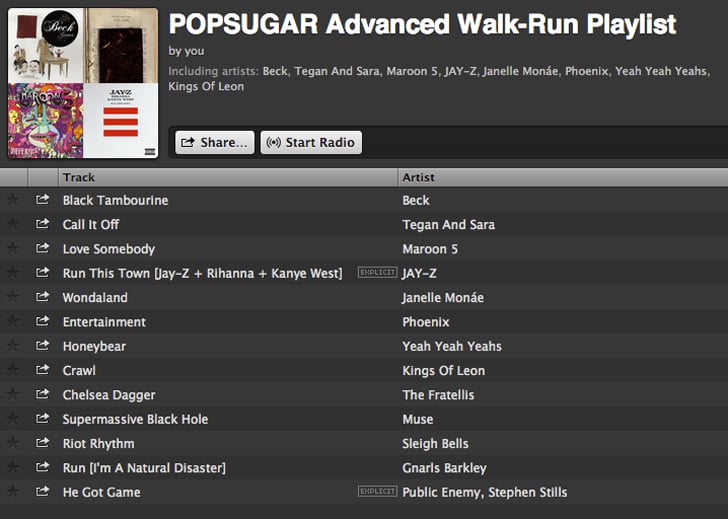A screenshot of an older version of iTunes displayed in a dark mode. The top left corner features an image collage of four album covers beneath a white text header that reads "Pop Sugar Advanced Walk One Playlist." Below, it mentions "by you," followed by a list of artists: Beck, Tegan and Sara, Maroon 5, Jay-Z, Janelle Monáe, Phoenix, Yeah Yeah Yeahs, and Kings of Leon.

Underneath the image, there are two buttons: one labeled "Share" and another marked "Starred Radio." The playlist details are shown in a table format. The first column displays star icons, all of which are unselected. The second column, presumably for sharing, also shows unselected white icons. The subsequent columns list the track titles and their respective artists.

The tracks included in the playlist are:
1. "Black Tambourine" by Beck
2. "Call It Off" by Tegan and Sara
3. "Love Somebody" by Maroon 5
4. "Run This Town" (explicit) by Jay-Z featuring Rihanna and Kanye West
5. "Wonderland" by Janelle Monáe
6. "Entertainment" by Phoenix
7. "Honeybear" by Yeah Yeah Yeahs
8. "Crawl" by Kings of Leon
9. "Chelsea Dagger" by The Fratellis
10. "Supermassive Black Hole" by Muse
11. "Riot Rhythm" by Sleigh Bells
12. "Run (I'm a Natural Disaster)" by Gnarls Barkley
13. "He Got Game" (explicit) by Public Enemy featuring Stephen Stills